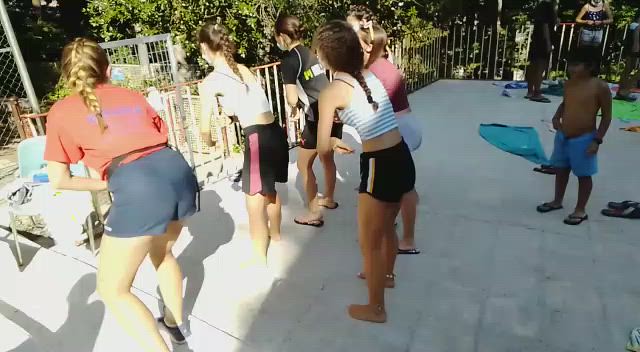The photograph captures a lively outdoor scene in broad daylight, set on a light-colored stone tile surface. Central to the composition is a group of young children, primarily girls, likely engaged in a dance routine or competition. Six girls are lined up, arranged in two rows with four in the front and two behind. They stand in coordinated poses, all facing to the left, their hair intricately braided and pulled back. Their attire consists of shorts and tank tops or t-shirts, and they are barefoot or in sandals. To the right of the group stands a younger boy in blue swim trunks and flip-flops.

Encircling the tiled area is a metal railing, providing a boundary to what seems to be a balcony or terrace. Brightly colored towels and scattered shoes are noticeable on the ground around the children. Beyond the immediate dance area, trees frame the top of the image, adding a natural, serene backdrop. In the shade, to the right, a few other individuals can be seen chatting and relaxing, adding to the sense of a communal outdoor gathering. The colors in the scene span a range of neutral and vibrant hues, including gray, tan, dark blue, maroon, light green, white, black, and lime green, contributing to the cheerful and dynamic atmosphere of the setting.